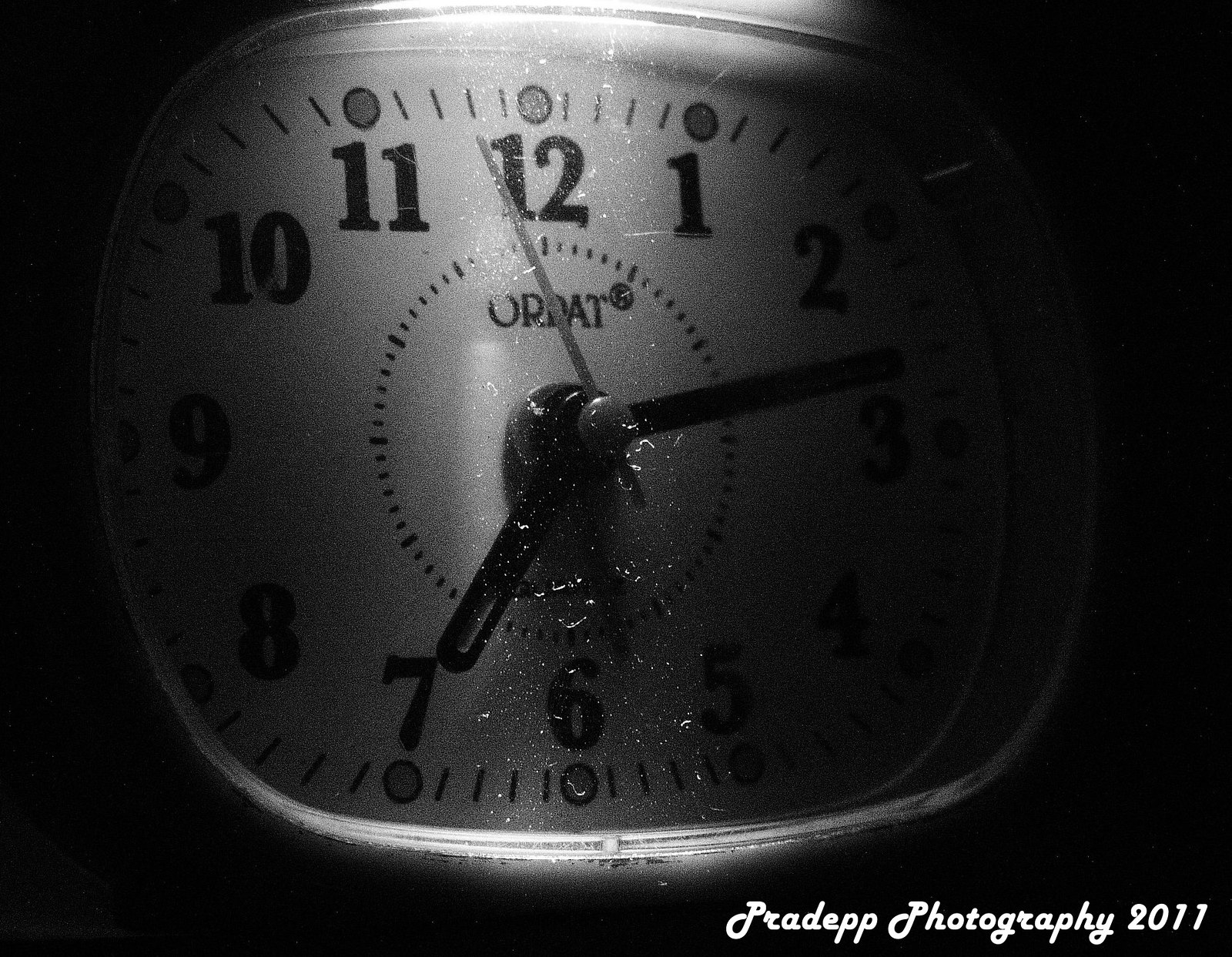This image features a striking clock face against a completely dark, black background. The clock face itself is white and is distinctly illuminated at the center top and center bottom. The clock is detailed with gray tick marks and circles outlined in black, each marking the hours. Beside each circle, the corresponding hour number is clearly displayed. Additional tick marks indicate the passage of seconds. In the center of the clock face is the word "ORDAT."

The clock has three hands: a thin gray hand for seconds, a shorter, thicker gray hand for minutes, and an even shorter, thicker black hand for hours. The bottom right corner of the image features the text "PRIDEP PHOTOGRAPHY 2011" in white, subtly indicating the photographer and the year the photo was taken.